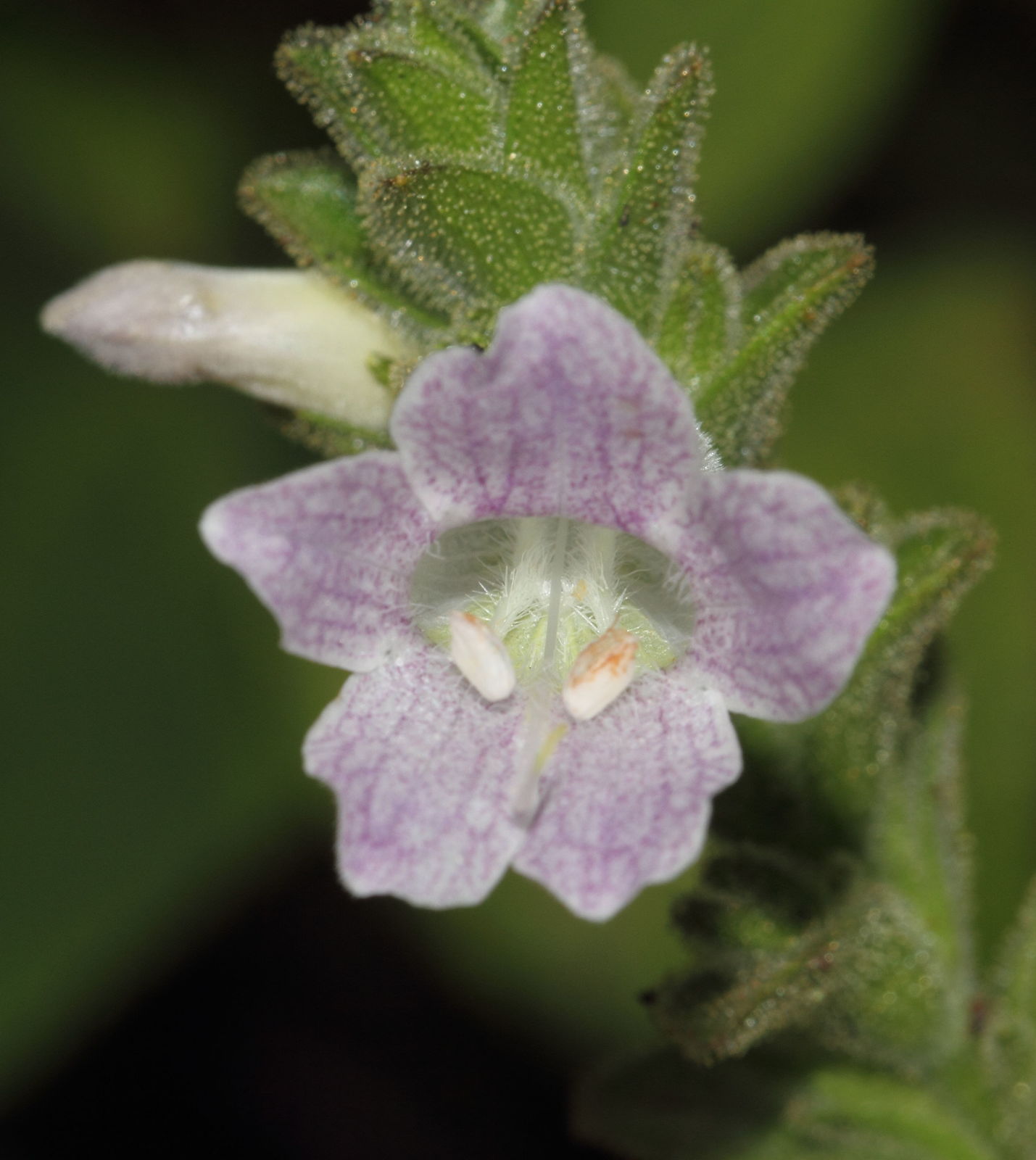The image captures a close-up, vividly detailed shot of a single flowering plant, possibly a nicotine plant. The flower dominating the frame is a delicate mix of light purple and white, forming a star shape with its five velvety, slightly fuzzy petals. Emerging from the center, two prominent white stamens tipped with a hint of orange add a textural contrast. Surrounding the flower are dense green leaves coated with tiny, sparkling trichomes that give them a hairy appearance. In the blurred background, another flower bud waits to bloom. The overall setting is brightly lit, enhancing the clarity and vividness of the scene, with the background fading to a mix of green and black to keep the focus on the intricate details of the flower and its immediate surroundings.